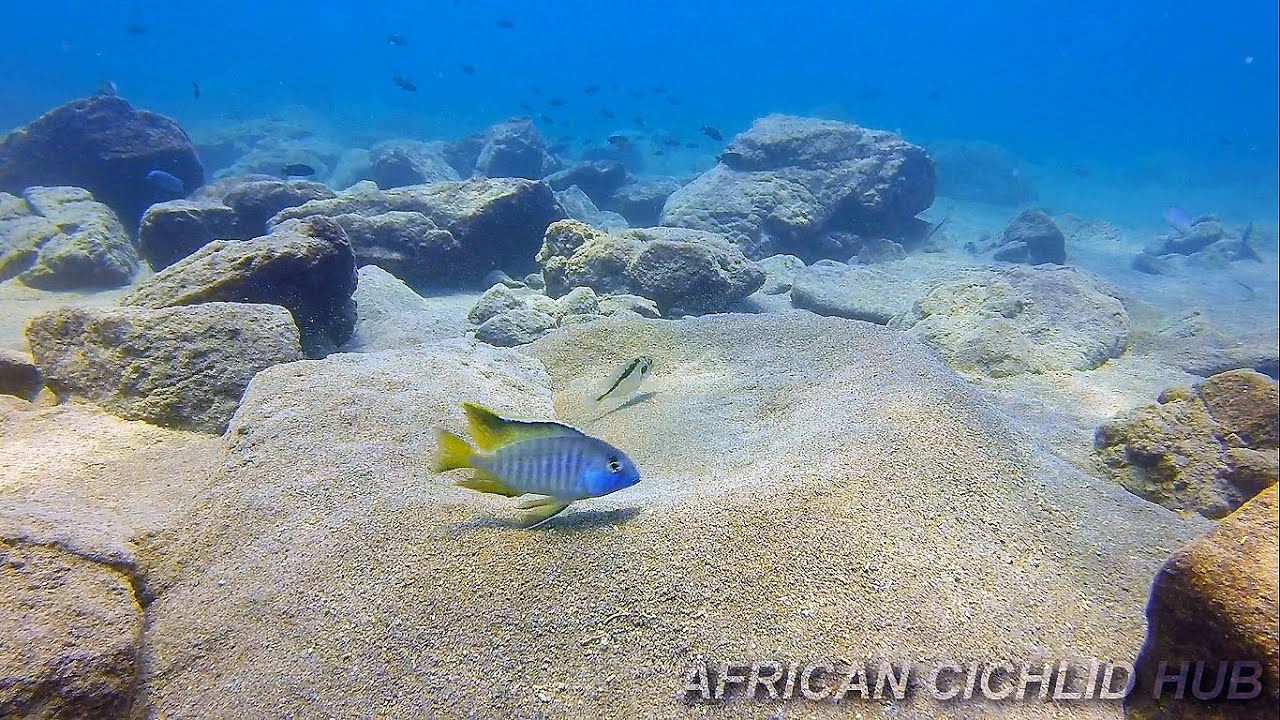This underwater tropical scene, marked by a translucent "African Cichlid Hub" watermark at the lower-right corner, showcases a stunning African Cichlid as the focal point. The fish, centrally positioned, boasts a light bright blue body adorned with vertical stripes, complemented by striking yellow fins and a yellow tail. A distinctive black mark runs through its eye, enhancing its exotic appearance. Surrounding the cichlid are large, boulder-like structures on a sandy seafloor. A transparent fish with a black line along its body can be seen just behind the cichlid. In the clear blue water background, schools of various fish swim amidst the underwater landscape, creating a dynamic and vibrant marine environment.